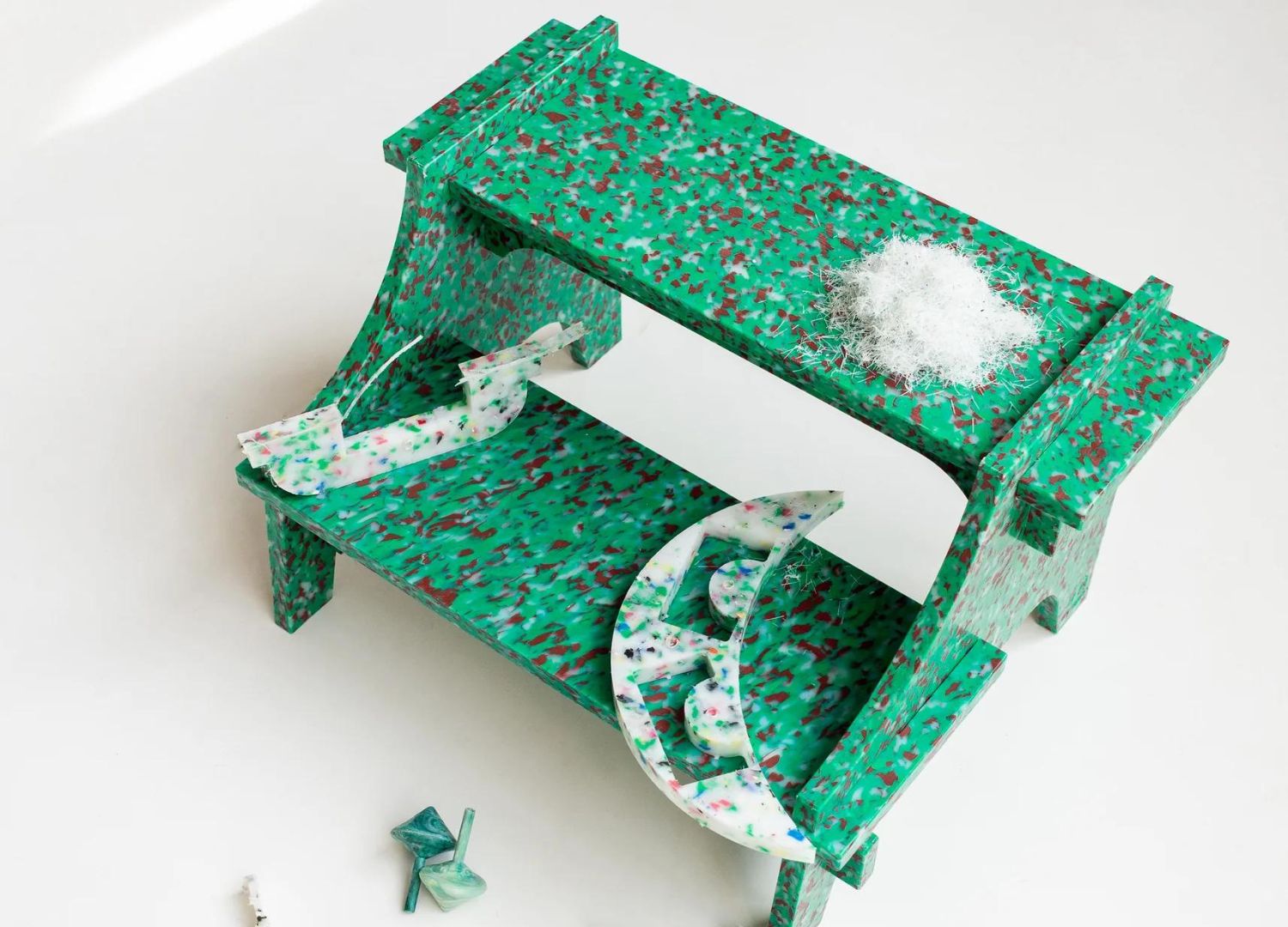The image displays a two-stepped structure, possibly an incense holder or step stool, crafted from a green material with a sheen, suggesting it might be painted wood. The surface is adorned with white and reddish spikes or dots. Positioned on a plain white background, the stool has the top step dusted with a white powder. The lower step features a crescent or cut-off moon shape, detailed with colorful dots in shades of white, blue, green, pink, and more, along with archways cut out of its inside. To the left of this shape, there is another white object, possibly an arch, also speckled with various colors. Additionally, two small, squarish knobs or pins are present at the bottom of the structure.